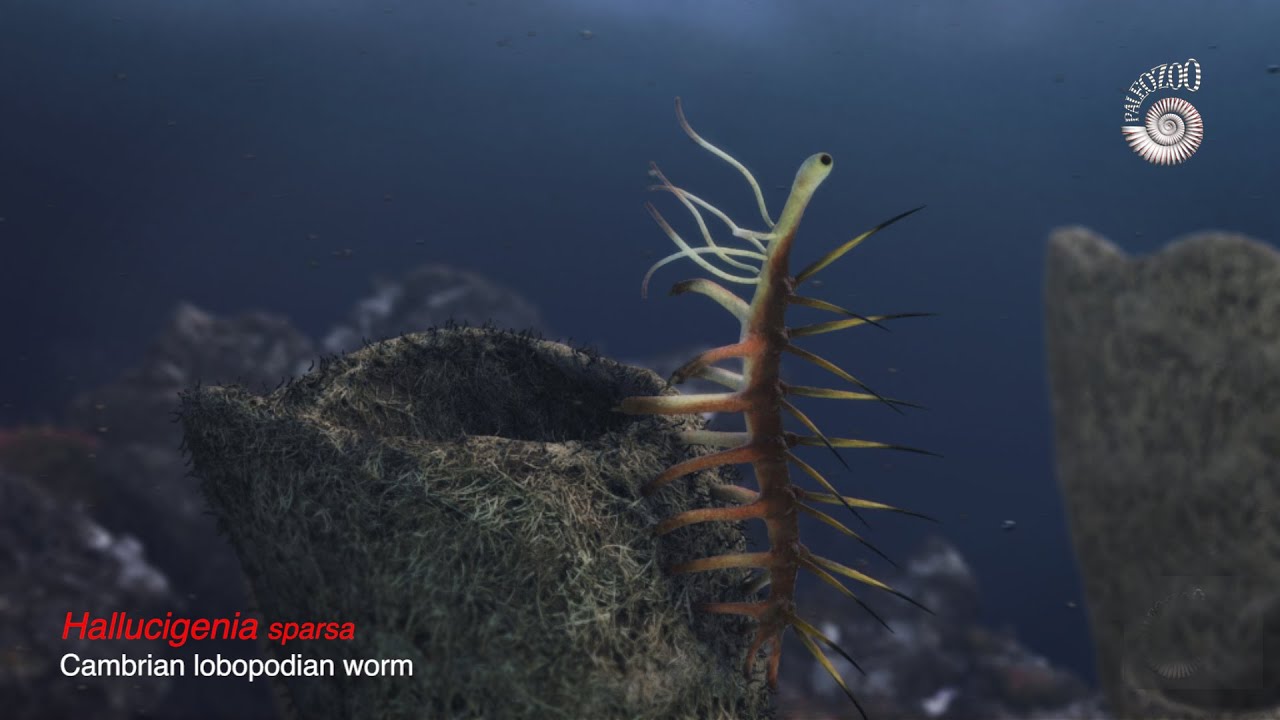The image is a detailed underwater photograph of a Hallucigenia sparsa, a Cambrian lobopodian worm. The background is a dark blue, evoking the depths of the ocean. The text "Hallucigenia sparsa" is displayed in red italics in the bottom left corner, with "Cambrian lobopodian worm" in smaller white font beneath it. The worm, orangish-yellow in color, has a thin, elongated body that is unique with numerous spiny appendages tipped in black. Its back features prominent spikes, while its head is equipped with what appear to be six wispy, antenna-like legs. The creature is latched onto a rocky, coral-like structure that seems to be covered in moss, creating a stark contrast between its vivid body and the textured, darker surface it rests upon. Paleozoo, perhaps indicative of the publication or exhibit, is labeled within the image, which adds to the scientific and paleontological context of this fascinating snapshot of ancient marine life.